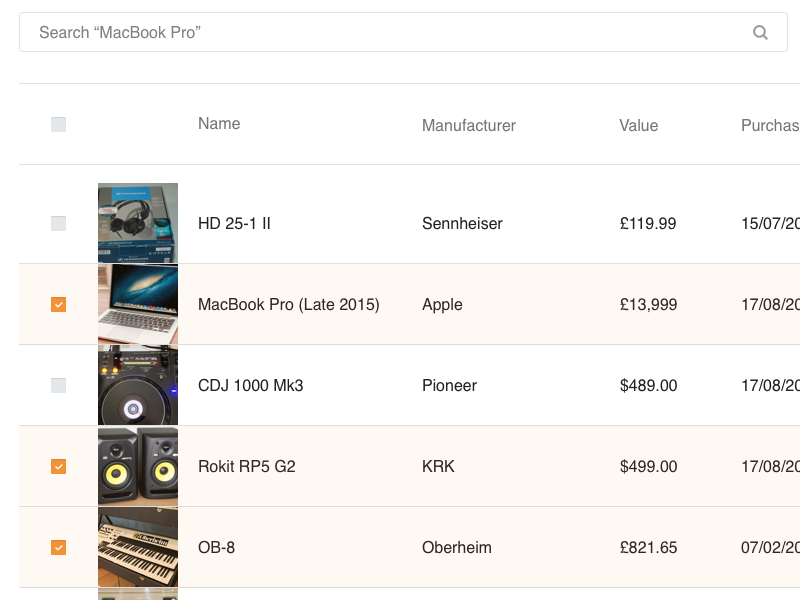The screenshot depicts the search results page on a MacBook Pro. At the very top, there is a prominently displayed search box with the phrase "Search MacBook Pro" highlighted within it. To the right of the search box is a small magnifying glass icon, which serves as the search button.

The search query "MacBook Pro" has been entered, generating five distinct results. Three of these results have been selected, indicated by a small orange box with a checkmark to the left of each image.

1. The first selected item is a "MacBook Pro Late 2015" by Apple, priced at 13,999 euros.
2. The second selected item is a "Rokit RP5G2" set of speakers, manufactured by KRK, priced at $499.
3. The third selected item is an "OB-8" synthesizer keyboard by Oberheim, priced at 821.65 euros.

The remaining two unselected items are a pair of headphones from Sennheiser and a DJ turntable from Pioneer.